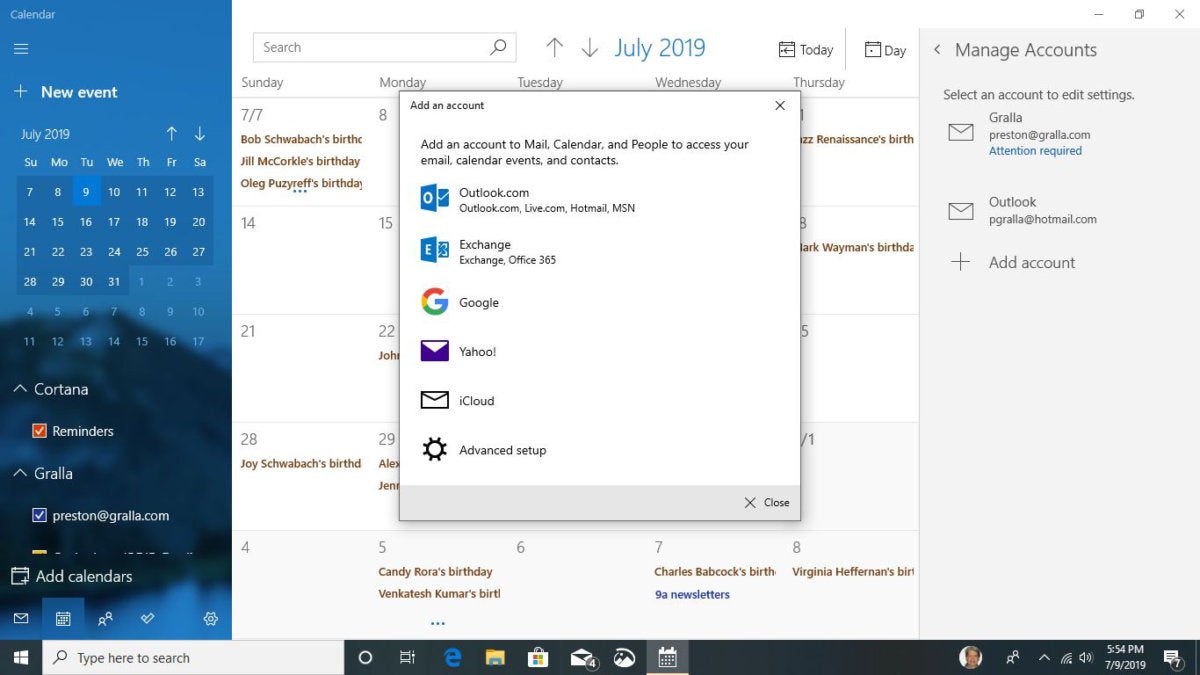Certainly! Here's a cleaned-up and detailed descriptive caption for the image described:

---

The image appears to show a Windows desktop screen with various UI elements and notifications. 

On the **bottom left**, there is a **Windows search bar**. Immediately to its right, there is a **circular icon** labeled with an "E," which presumably stands for Microsoft Edge. Next to Edge, there's a **folder icon** followed by the **Microsoft Store** icon. Moving further right, the symbols include a **letter icon** and a **number 4** at the far bottom right corner.

In the **bottom right**, there are several icons including a **calendar** and **photo thumbnails**. Above these, there's a row of additional symbols which include a **speaker icon**, and the time displayed as "5:54 PM". Alongside, there is a sequence of numbers "7-9-7-7-18", possibly representing messages or notifications.

On the **top left corner**, there's a Calendar application open titled "Post New Event", showing **July 2019**. Just below, there is a mention of **Cortana** and a reminder note with "Gorilla, Preston, and Gorilla.com".

To the **far right of the screen**, there is a section for managing accounts, such as "Select accounts and settings" with the names **Gorilla, Preston, and Gorilla.com** listed. This is followed by options like "Send a sales ad account," "Add an account to mail," "Calendar people," "Email account," "Add to contact," and services like **Exchange, Google, Yahoo, iCloud**, and **Advanced setup**.

In the background, a calendar possibly lists several birthdays and events: "Bob's," "Charlotte's birthday," "Jill McCork's birthday," "Ola's birthday," "Joy's," "Charlotte's birthday" (repeated for emphasis), "Kendi Roa's birthday," "Vin Katesh Kumar's birthday," "Charles Bemkock's birthday," and "Virginia Hefferman's birthday". There is also a mention of "90 newsletters."

---

I hope this helps! If you have more specific details or additional context for any part of the descriptions, let me know, and I can refine it further.